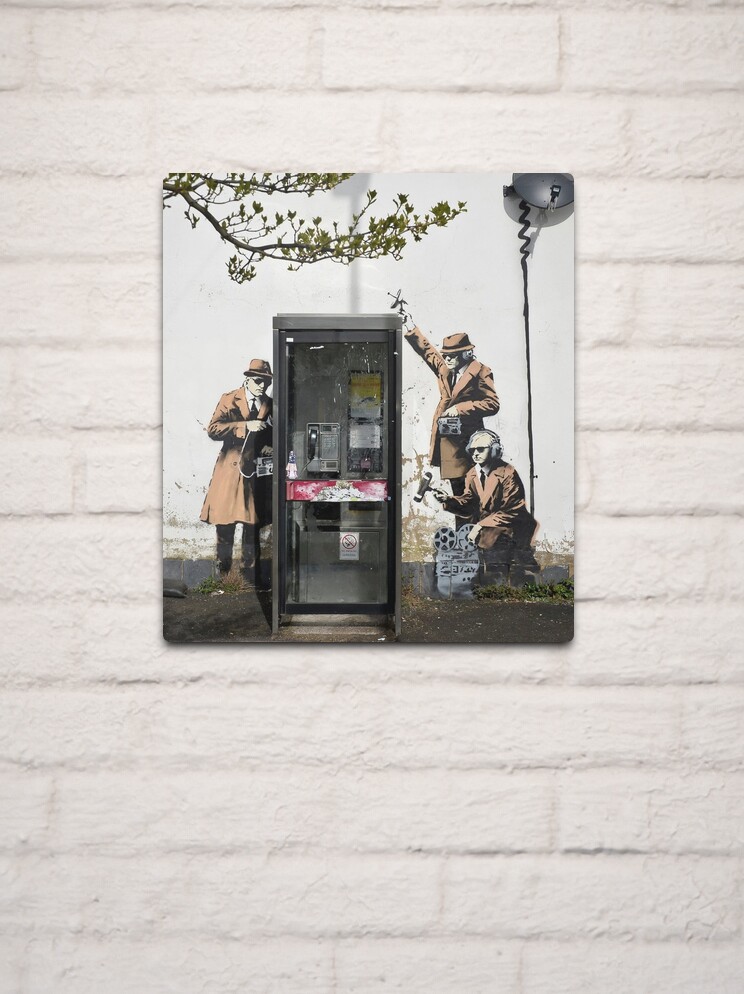On a white brick background, painted in clean white, hangs an intricate art piece depicting an old-fashioned black telephone booth with a glass door. Surrounding the booth are three men, all dressed in brown trench coats and hats, reminiscent of spies or FBI agents. The man on the left, who has a receding hairline, is kneeling next to the phone booth, possibly holding a can of spray paint or a paint roller, with a cinematic film roll by his side. Behind him, another gentleman in a long trench coat and hat stands with a spy antenna pointing skyward. On the opposite side, the third man, also in a trench coat and hat, leans against the booth, wearing glasses. The men seem to be engaged in a surveillance operation, using various equipment to eavesdrop or analyze the booth, conveying a sense of intrigue and mystery. Overhead, a green-leaved tree branch adds a touch of natural contrast against the otherwise stark background. This detailed artwork captures the essence of a bygone era with a hint of cinematic suspense.